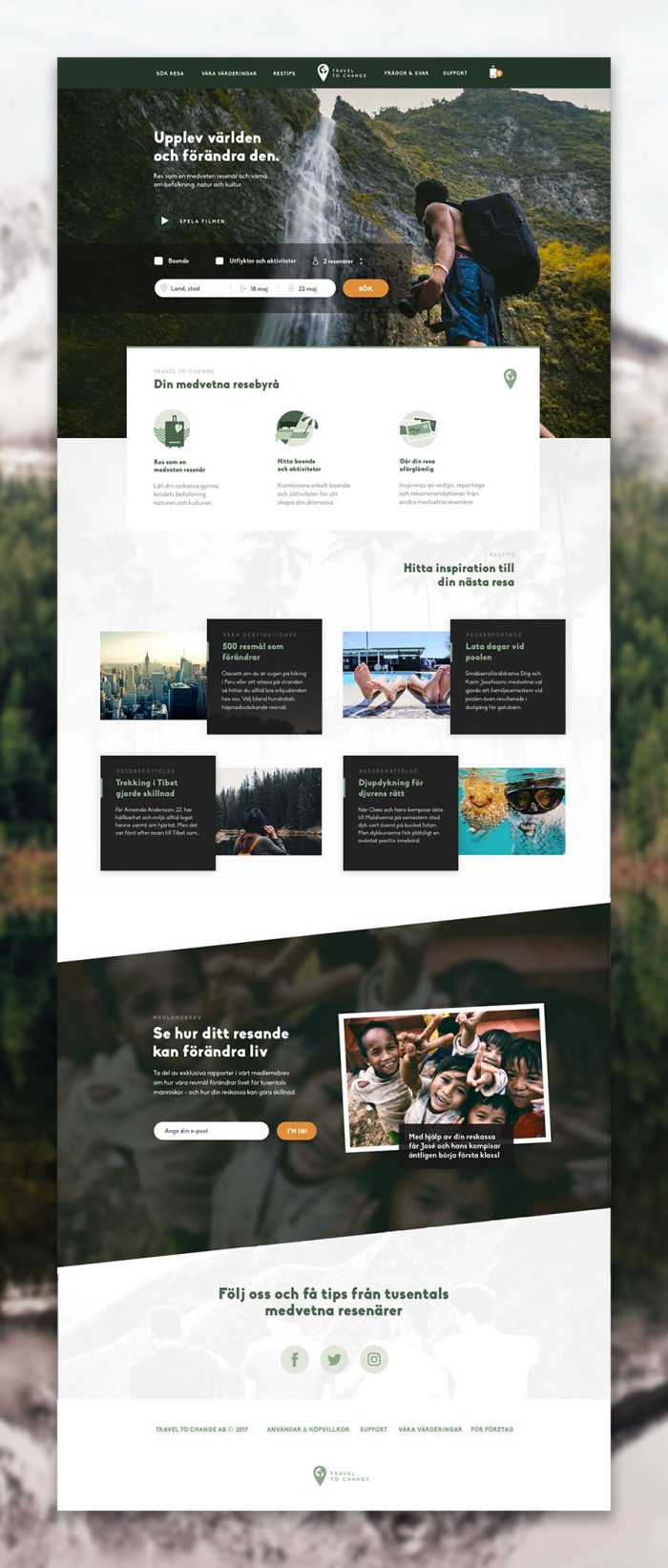The image is a tall, narrow, vertical advertisement, likely a window display or digital brochure, featuring multiple layers of content. At the top is an image of a man standing in front of a majestic waterfall cascading down a mountain, with some white text next to him that's too small to read. Below this, there are overlapping advertisements presented on a white background. One section includes three columns of text, each starting with indistinct graphics followed by bold headlines and lighter text. Another section showcases a grid of eight square panels, alternating between photographs and black text boxes. The photos depict a cityscape, a resort scene with people by a pool or beach, a mountain with a lake, and hot air balloons in the sky. Additional advertisements feature columns of text, bold white letters on a black background, and a picture of a cheerful family at a resort. At the very bottom, there are logos for Facebook, Twitter, and Instagram, and some centered black text on a white background, too small to read. The final line of text reads "Travel to change," accompanied by a location icon.